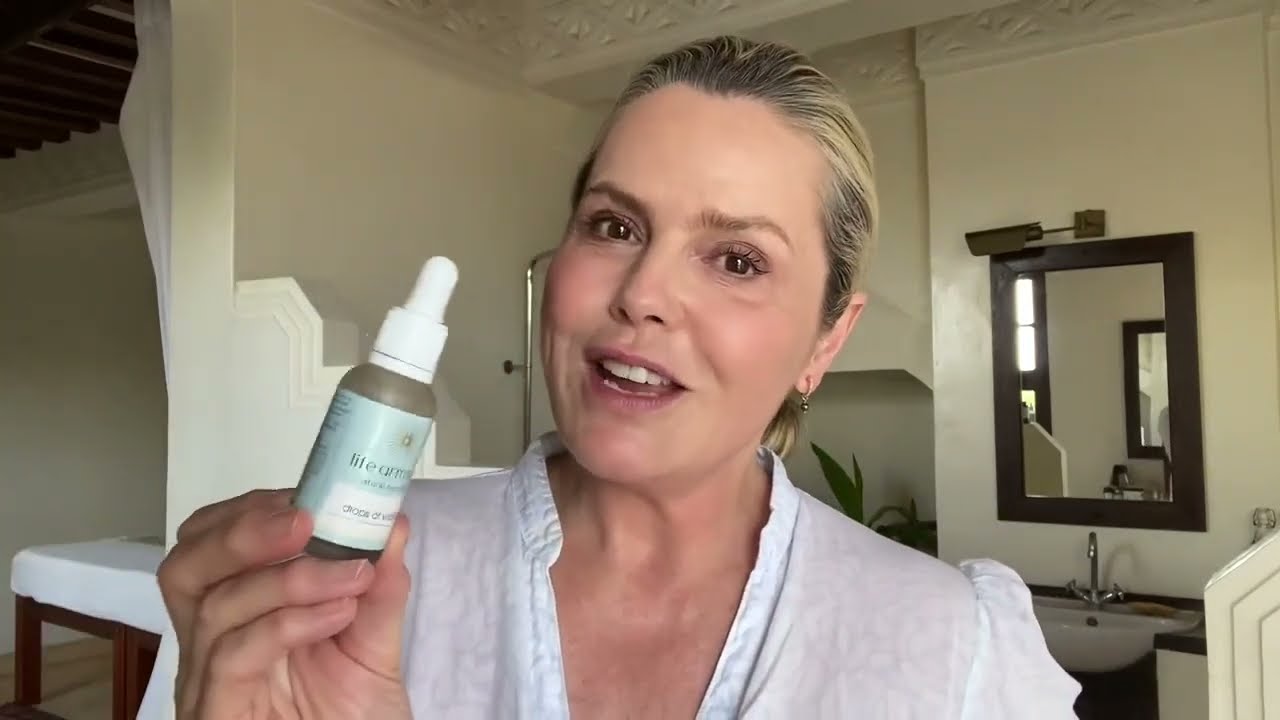In this horizontal, landscape-oriented color photograph, a woman in her late 30s or early 40s is the central focus. She has light skin and blondish hair with brown highlights, pulled back in a ponytail or bun. Her light blonde streaked hair frames her face, where she has brown eyes accentuated with mascara. Small beaded earrings adorn her ears, complementing her white V-neck blouse. 

The woman, who is speaking, holds up a green bottle with a white drop dispenser cap in her right hand, prominently displaying its light blue label with an illegible logo and text. The setting appears to be a bathroom or spa-like environment; behind her, a dark brown framed mirror hangs above a sink basin with a silver faucet. A green potted plant peeks from her shoulder, adding a touch of nature to the scene. The greenish-colored walls and a visible light fixture contribute to the cozy, home-like atmosphere. To the left of the sink, an opening reveals an adjacent room featuring a dark wood massage table covered with a white cloth, and exposed beamed ceilings complete the tranquil setting.